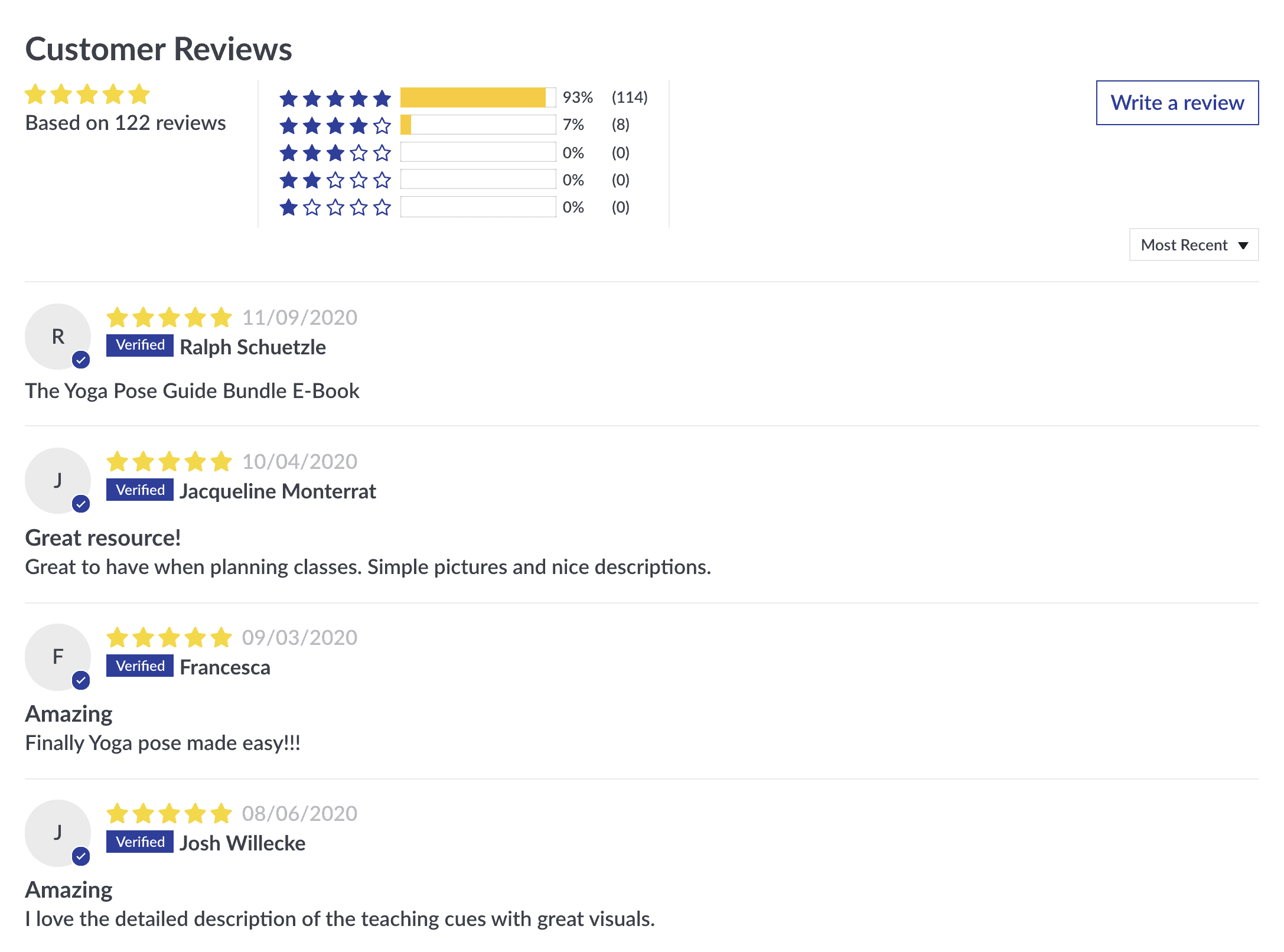**Image Description: Customer Review Overview – Detailed Breakdown**

At the top of the page, the title "Customer Reviews" is prominently displayed. Accompanying this heading is a visual representation of five yellow stars, indicating an average rating. It specifies that the rating is based on 122 reviews. To the right of this section, a detailed breakdown of the ratings is presented in bar and numeric formats:

1. **Five Stars:**
   - Percentage: 93%
   - Number of Reviews: 114
   - Represented by a yellow bar

2. **Four Stars:**
   - Percentage: 7%
   - Number of Reviews: 8
   - Represented by a green bar

3. **Three Stars:**
   - Percentage: 0%
   - Number of Reviews: 0

4. **Two Stars:**
   - Percentage: 0%
   - Number of Reviews: 0

5. **One Star:**
   - Percentage: 0%
   - Number of Reviews: 0

On the right end of this section, there is a prominent yellow rectangular button labeled "Write a Review."

Immediately below this analysis, there is a section labeled "Most Recent" with a downward-facing triangle, likely indicating a dropdown menu or filter option.

Following this, four individual reviews are listed in sequence:

1. **Review by R (Ralph Schutzel):**
   - Icon: Circle with a checkmark
   - Rating: Five stars
   - Date: 11-09-2020
   - Status: Verified
   - Comment: "The Yoga Pose Guide Bundle eBook."

2. **Review by J (Jacqueline Monerat):**
   - Icon: Circle with a checkmark
   - Rating: Five stars
   - Date: 10-04-2020
   - Status: Verified
   - Comment: "Great resource, great to have when planning classes. Simple pictures and nice descriptions."

3. **Review by F (Francesca):**
   - Icon: Circle with a checkmark
   - Rating: Five stars
   - Date: 09-03-2020
   - Status: Verified
   - Comment: "Amazing, finally Yoga Pose Made Easy."

4. **Review by J (Josh Wilicki):**
   - Icon: Circle with a checkmark
   - Rating: Five stars
   - Date: 08-06-2020
   - Status: Verified
   - Comment: "Amazing. I love the detailed description of the teaching cues with great visuals."

This structured layout provides users with a comprehensive view of product feedback, enabling informed decision-making.